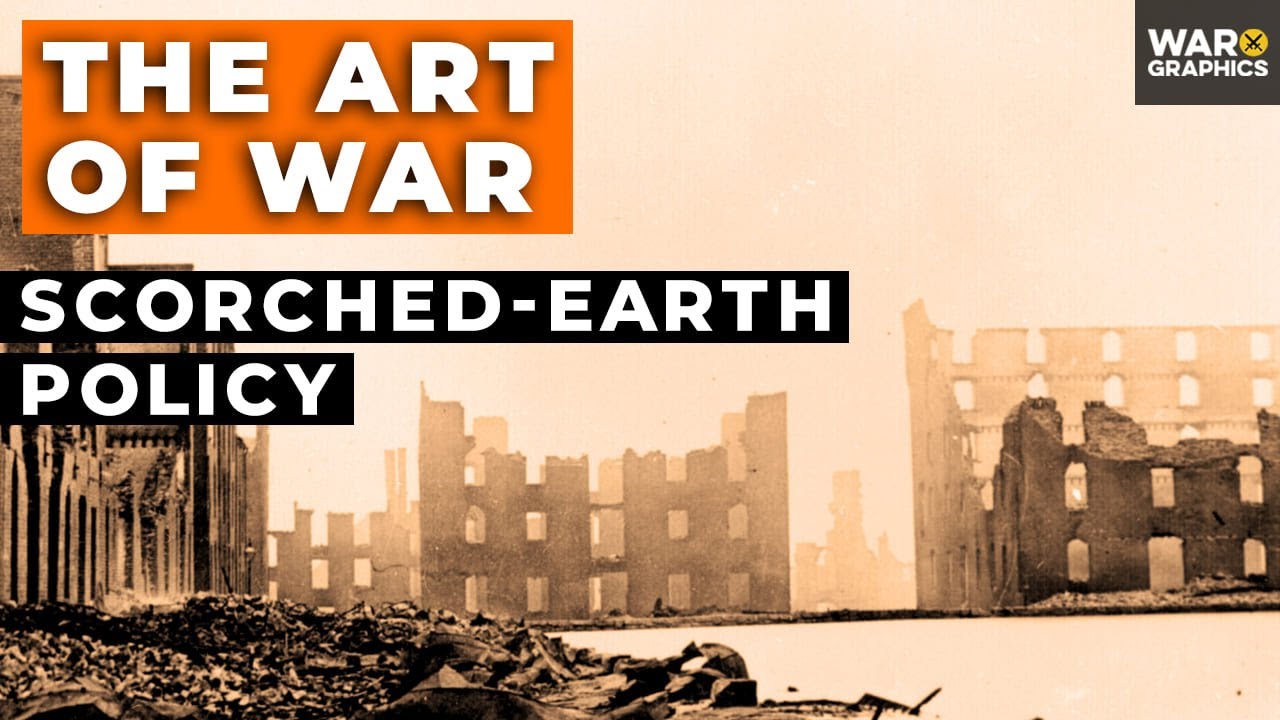This is a black and white poster with a very light peach background, depicting a bombed-out cityscape. The scene is dominated by crumbling buildings, shattered at various floors, and piles of rubble scattered across the foreground. An orange-yellow haze envelops the entire city, adding to the desolate atmosphere. 

In the upper left corner, there is a dark orange text box with white letters that read "The Art of War, Scorched Earth Policy." The phrase "Scorched Earth Policy" appears again in large capital white letters on a black background. In the upper right corner, a smaller gray text box with white letters states "War Graphics," accompanied by an image of two crossed swords over a yellow background. This imagery and text suggest the poster might be the cover of a picture book, report, or screenplay focusing on the devastation caused by war and the scorched earth tactics employed.